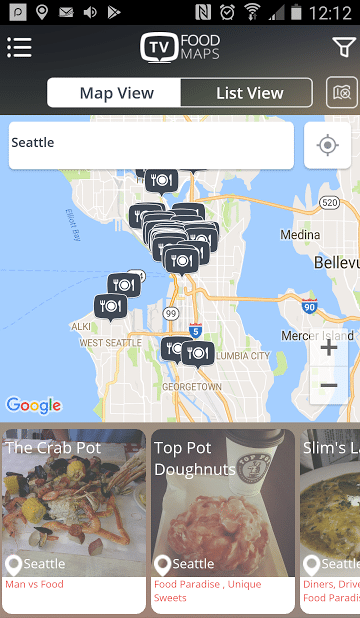A smartphone screen displays a detailed map of Seattle. At the top, the status bar shows icons for a strong wireless signal, a nearly full battery, and the current time marked as 12:12. Directly below, three tabs labeled "TV," "Food," and "Maps" are visible, with "Map View" highlighted and "List View" as an alternative option.

Below this interface, the map of Seattle is prominently shown, marked with various icons indicating points of interest. Many of these icons represent restaurants, identified by symbols of a fork, a plate, and a knife, though none are labeled with specific names.

At the bottom of the screen, the word "Google" appears above a row of food-related images. The first image on the left, labeled "The Crab Pot," displays a dish from the restaurant and includes the text "Man vs. Food." The second image shows a coffee cup with the "Top Pot" logo and a donut, labeled "Top Pot Donuts," along with mentions of "Food Paradise" and "Unique Sweets." Both pictures also feature the word "Seattle" prominently.

This screen provides a comprehensive view of Seattle's map and highlights local dining options with visual and textual details.